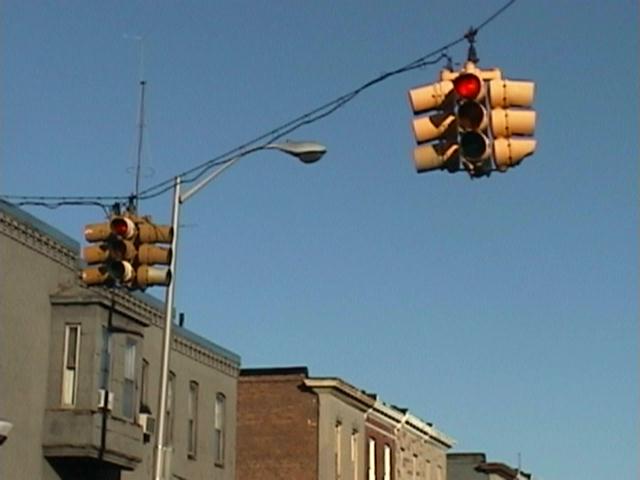The image showcases a clear and vibrant robin's egg blue sky, devoid of any clouds. Suspended prominently in the air by black cables, two yellow traffic lights are visible, each displaying a red signal. The cables form an arc, starting approximately 30% from the right of the top edge, swooping down, and reattaching about 40% down the left side. One traffic light hangs around 15% from the start of the cable, while the other is positioned about 20% from the left.

The traffic lights are designed with four sides and feature tubes to ensure visibility from specific angles. A large metal streetlamp is also visible near the center of the image.

Below the suspended lights, the upper stories of several buildings line the scene. On the lower left, there is a gray building, beside which stands a brick building followed by a tan building. Additional details include a large antenna atop the closest gray building and another metal pole emerging from a distant building. The setting evokes a small town's downtown area, with buildings likely accommodating both residential and commercial spaces.